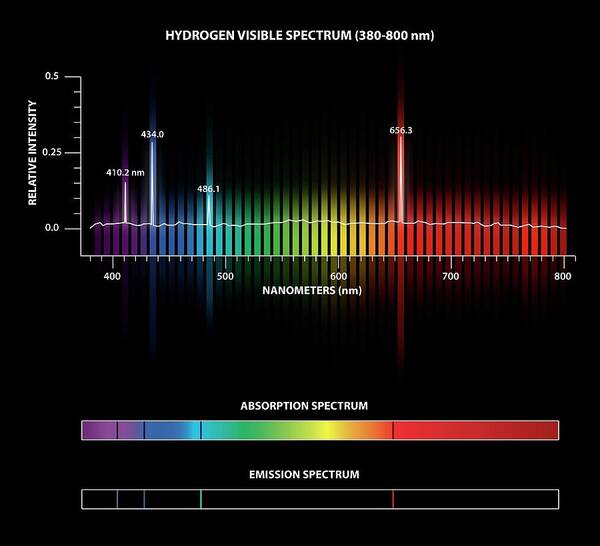The image is a scientific chart, set against an all-black background, detailing the hydrogen visible spectrum from 380 to 800 nm. At the top, in white writing within parentheses, it reads "hydrogen visible spectrum 380-800 NM." The chart is segmented into colors reminiscent of the rainbow—including purple, blue, green, yellow, orange, and red. The x-axis, labeled "nanometers," ranges from 400 to 800 NM, while the y-axis, marked "relative intensity," scales from 0 to 0.5. 

Specific values are highlighted with spikes at 410.2 nm (purple), 434 nm (blue), 486.1 nm (turquoise), and 656.3 nm (orange). Below the primary graph, there is an "absorption spectrum," represented by a bar transitioning through the same rainbow colors, with green, yellow, orange, and red being the most prominent, while purple and blue are the smallest. Further down, an "emission spectrum" features another bar adorned with distinct thin lines in white, turquoise, and red.